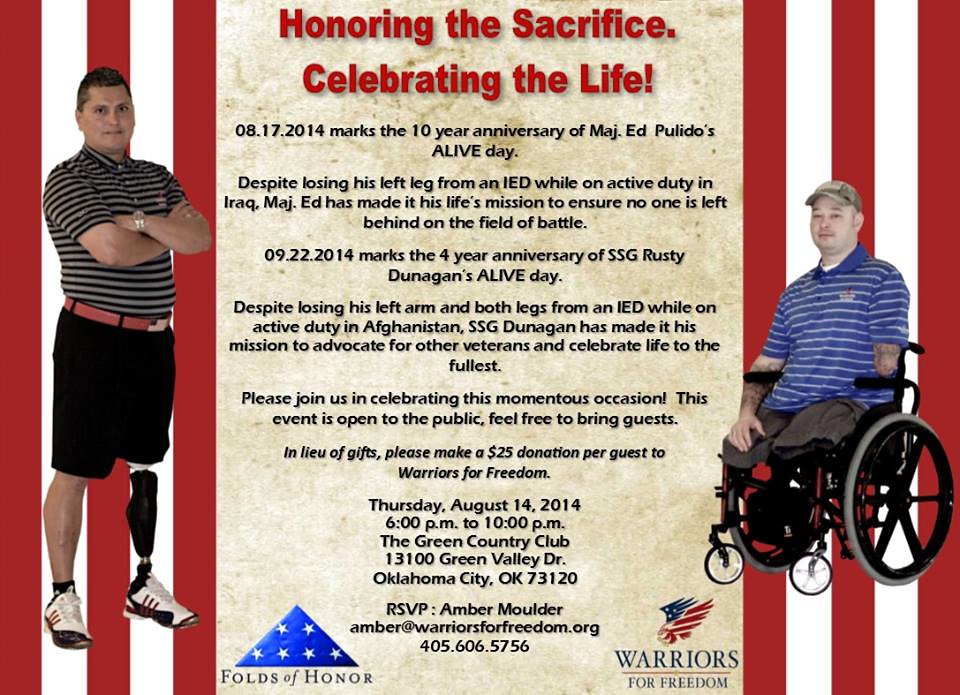The image features a visually impactful, digitally designed tribute poster. It has a backdrop with vertical red bars on either side, three on each side. In the center, in bold red letters, it says "Honoring the Sacrifice, Celebrate the Life." The background behind the text is a textured, dirty beige color with black text on it.

In the foreground, two men are depicted. One man, standing, has short black hair, wears a polo shirt and black shorts, and has one prosthetic leg. The other man is seated in a wheelchair, wearing a cap and blue shirt; he has one arm and no legs.

The text informs viewers that August 17, 2014, marks the 10th anniversary of Major Ed Toledo's 'Alive Day,' despite him losing his leg due to an IED in Iraq. It also mentions that September 22, 2014, is the 4th anniversary of SSG Donnegan's 'Alive Day,' following the loss of his left hand and legs from an IED in Afghanistan. Both veterans have dedicated their lives to advocating for other veterans.

Icons of the Folds of Honor, a triangle American flag, and the Warriors for Freedom logo are present at the bottom right of the poster. The event details are also provided: Thursday, August 14, 2014, from 6 to 10 PM at Green Country Club, 1300 Greenvale Drive, Oklahoma City, Oklahoma, 73120. The event is open to the public with a suggested donation of $25 per guest to Warriors for Freedom. RSVP details include an email to Amber at warriorsforfreedom.org and a contact number, 405-606-5756.